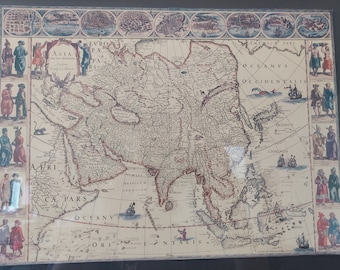This image displays an ancient, hand-drawn map, possibly mounted on a dark gray or black wall. The square map is intricately detailed, featuring a full-color print with borders along the top, right, and bottom. The borders are segmented into small squares, five on each side, each containing two people dressed in alternating blue and brown outfits. In addition, there are oblong shapes along the top, embedded with designs, totaling nine in number.

Filling in the map's center are depictions of various sea monsters and ships navigating the ocean, rendered in brown and tan hues. The background is light tan, and though there is text scattered throughout, it is too small to be legible. At the top of the image, nature scenes are faintly visible. The map, adorned with minute imagery and possibly historical icons, is surrounded by detailed miniatures of people and possibly symbolic figures, making it a richly ornate and enigmatic artifact.